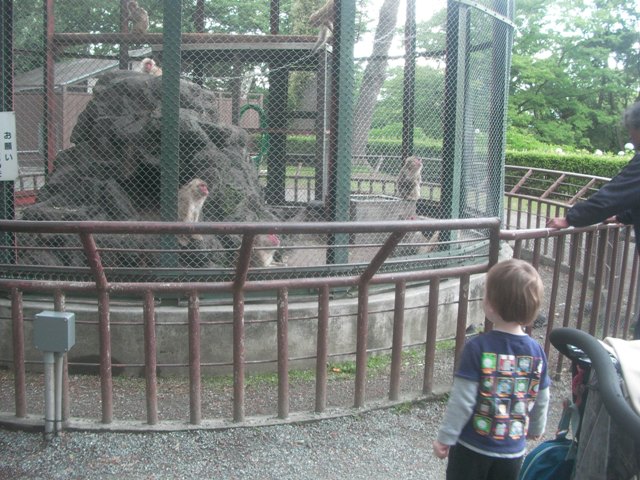In the bottom right-hand corner of the image, there's a toddler with short light brown hair, facing away from the camera. He is wearing a graphic t-shirt with a design that looks like Thomas the Train and friends, layered over a long-sleeved gray shirt. Black pants complete his outfit. Nearby, partially cut off on the bottom left-hand side, the handle of a stroller is visible.

The main focus of the photograph is a circular zoo exhibit surrounded by a rusted red and light brown round metal fence. A person with dark sleeves is seen leaning on this fence on the right side of the image. Inside the enclosure, green metal supports hold up a chain mesh fence. 

Central to the exhibit is a large gray rock formation with small monkeys climbing atop and around it. These monkeys have gray fur and distinctly pink faces. The photo captures the playful environment within the exhibit, as the monkeys move about their habitat.